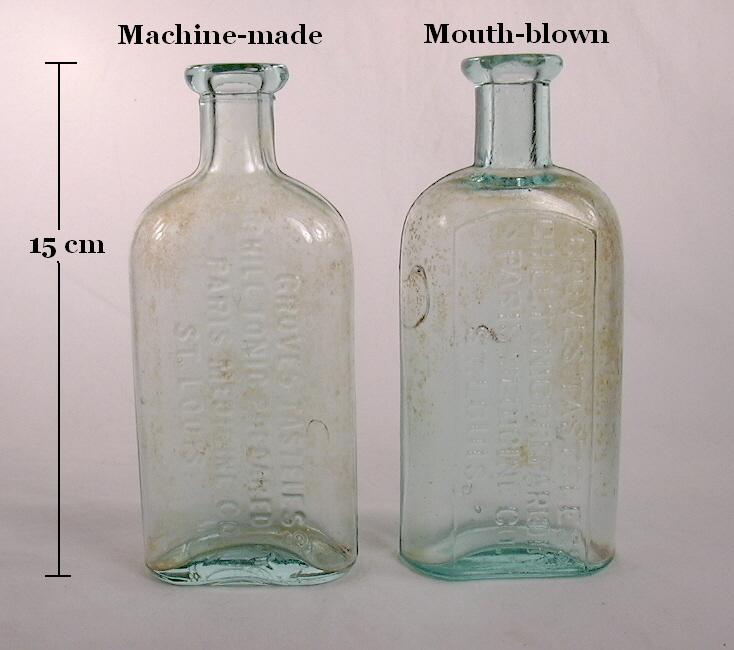This photograph presents a side-by-side comparison of two vintage glass bottles, both standing on a light gray surface with a matching background. Each bottle is 15 cm in height, confirmed by the scale marker positioned on the left. The bottle on the left is identified as machine-made, while the bottle on the right is labeled as mouth-blown. 

Both bottles share a similar structure with wide bodies, skinny necks, and round openings, but the mouth-blown bottle exhibits a more irregular shape with wider, rounder shoulders and a crooked neck. The machine-made bottle appears more uniform but still slightly off-kilter at the base. Each bottle shows signs of age, including a brown tinge indicative of grime or dust accumulation and small bubbles trapped in the mouth-blown glass. Despite their vintage construction and evident wear, the inscriptions on the glass remain difficult to read due to the clear material and light penetration.